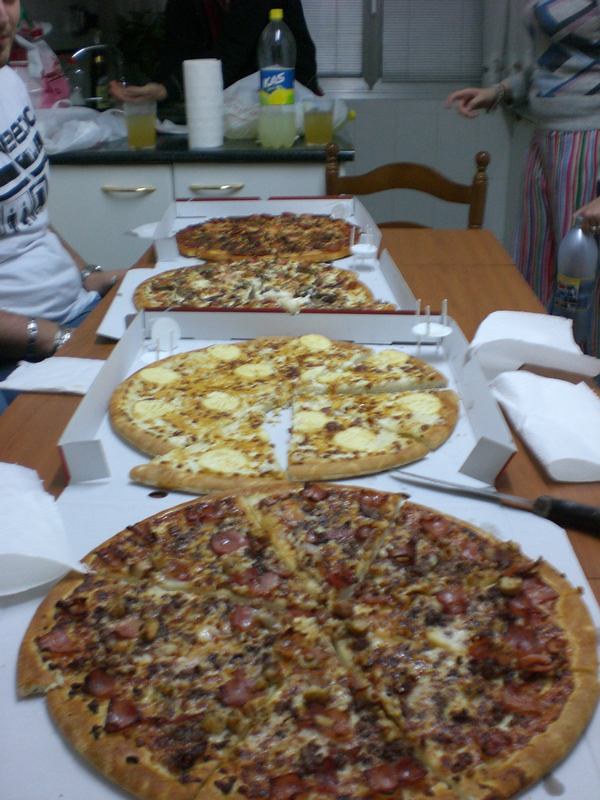In this image, we observe a casual pizza gathering featuring four distinct pizzas, all arranged in a row on opened pizza boxes to protect the wooden table. The pizzas vary in toppings: the closest pizza sports a light brown crust with pepperoni and perhaps other meats, while the second pizza is a white cheese pizza. The other two pizzas further out appear to have a combination of cheese, bacon, and mushrooms, each adorned with white separators in the middle. The pizzas rest on parchment paper atop the opened boxes.

In the background, a black countertop with white drawers and gold handles is visible, housing a clear plastic bottle labeled "KAS," a roll of paper towels, and two cups. A person wearing a grey top and red and blue checkered pants stands pointing forward, while another person sits off to the left, wearing a white T-shirt with black lettering. Toward the right of the image, there's a wooden chair with round spindles and a knife with a black handle on the table, along with strewn white napkins.

The scene conveys a friendly atmosphere with ample provisions for everyone, such as beverages and paper towels for easy clean-up. The setting, complete with venetian blinds over a window and an empty chair at the table, enhances the cozy, inviting vibe.